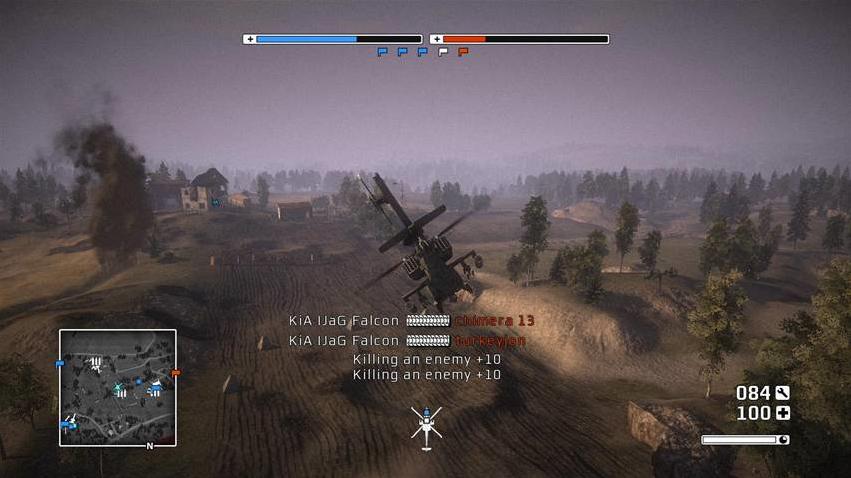This screenshot from a highly realistic video game depicts a military helicopter soaring above a vast expanse of farmland. The detailed graphics create an immersive atmosphere, showcasing an expansive landscape with significant empty plains and a scattering of trees, primarily concentrated on the right side of the image. In the distant background, a dense forest fringes the horizon, interspersed with a singular building that appears to be the source of a billowing plume of smoke, possibly indicating a recent target strike. In the lower left corner of the screen, an aerial map provides an overview of the current location, complete with icons suggesting the positions of other helicopters. Across the top of the image, two meters—colored blue and red—offer vital gameplay information, while text at the bottom center of the screen notifies players of enemy combatants being killed.